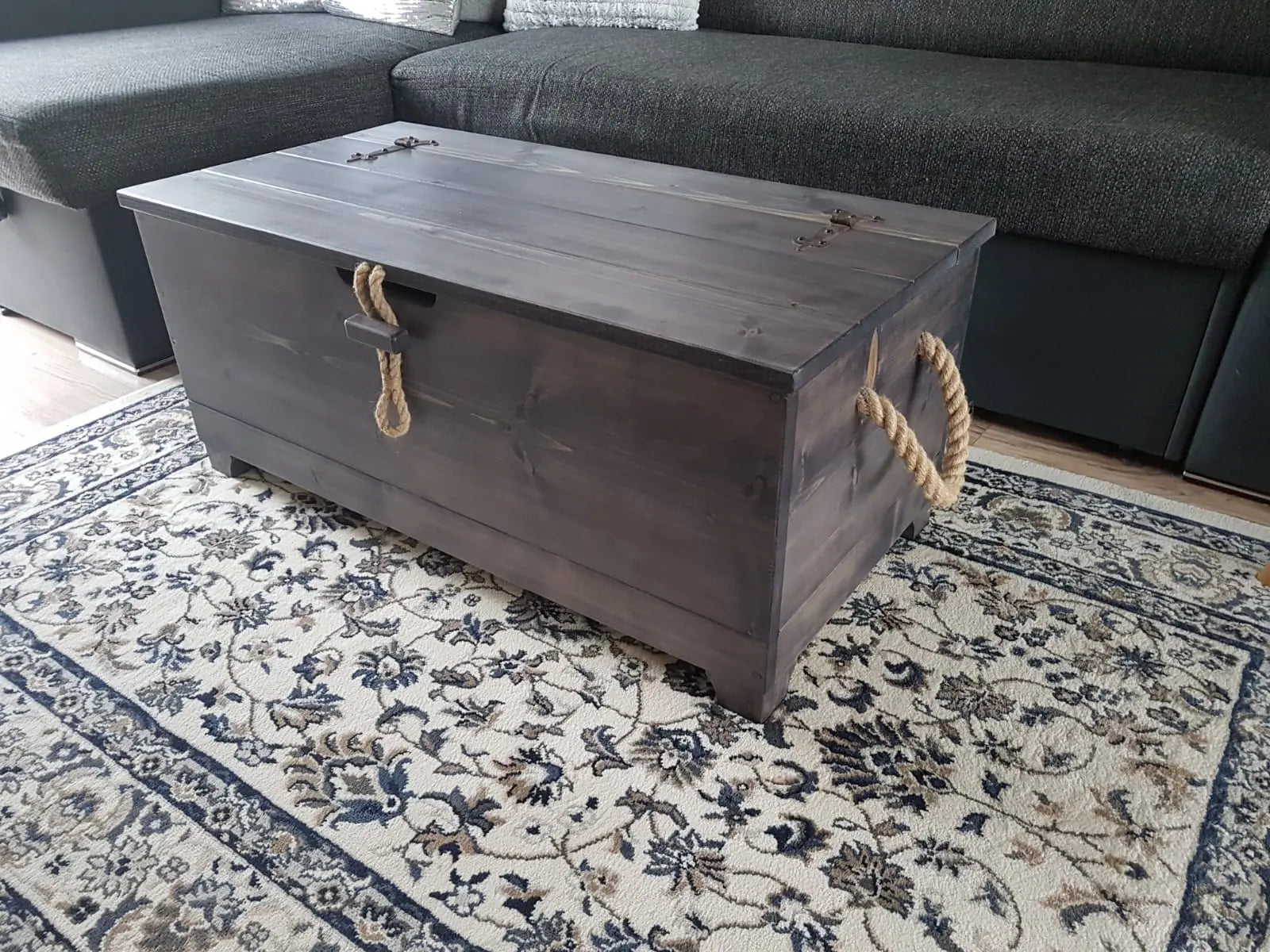This image captures a cozy living room scene featuring a large, dark wooden chest that serves as a coffee table. The chest, occupying about 50% of the image, is slightly off-center to the left. Made from heavy, dark-stained wood featuring a satin finish, it has a rustic aesthetic with nailed slats forming its top and sides. The chest is equipped with two brown metallic hinges on the lid, a light brown rope handle on one end, and another piece of rope at the front acting as a latch. It stands on four small feet and rests atop a detailed, ornate rug with a predominantly white background adorned with intricate floral designs in blue, brown, and olive tones. The living room setting includes a sectional sofa behind the chest, composed of dark gray or black fabric and leather, with two visible pillows—one silver and one white. A glimpse of light brown hardwood flooring can be seen around the edges of the rug, adding a warm touch to the room's decor.